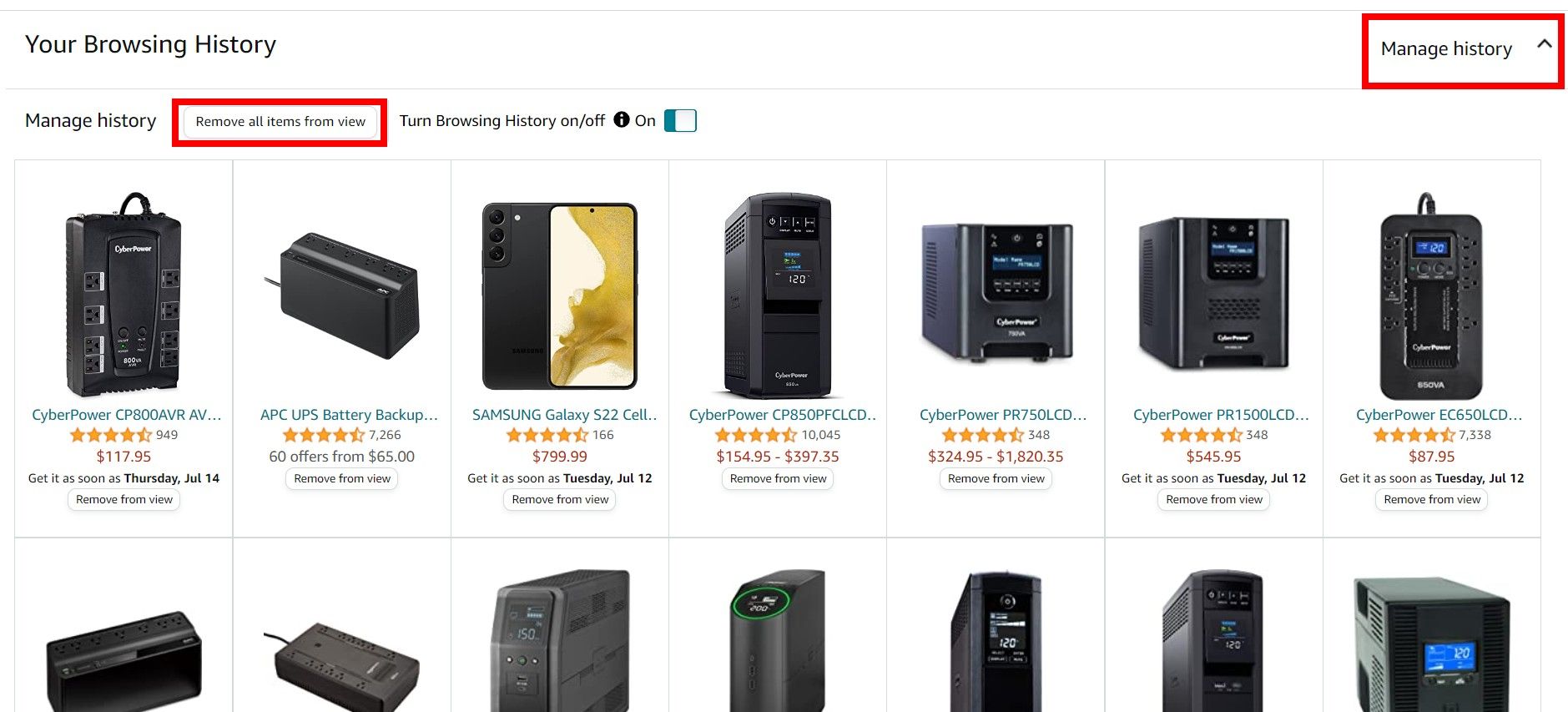This screenshot captures a user's browsing history page. At the top left corner, bold text proudly announces, "Your Browsing History." Oppositely, in the upper right corner, "Manage History" is highlighted within a red border. On the left side of the page, "Manage History" appears again, adjacent to another red-bordered option titled "Remove All Items from View." Below, the phrase "Turn Browsing History On/Off" is accompanied by a filled-in dot next to "On." 

The main content showcases images and descriptions of seven items stretched across the page. The first item is a black rectangular object labeled "CyberPower CP800AVRAV..." followed by a star rating, number of reviews, and the price: $117.95. It offers expedited shipping with, "Get it as soon as Thursday, July 14," and includes an "Remove From View" option beneath it.

To the right, another black rectangular item is identified as "APC UPS Battery Backup," with "60 offers from $65.00." The third item is a phone, "Samsung Galaxy S22," followed by multiple CyberPower products: "CyberPower CP850P" and similar items. The issue continues with a series of related CyberPower devices.

Below the first row, a second row of seven products, all black and electronically related, is partially obscured. Only the top parts of these products are visible, while the text beneath them is cut off, providing an incomplete view of the items.